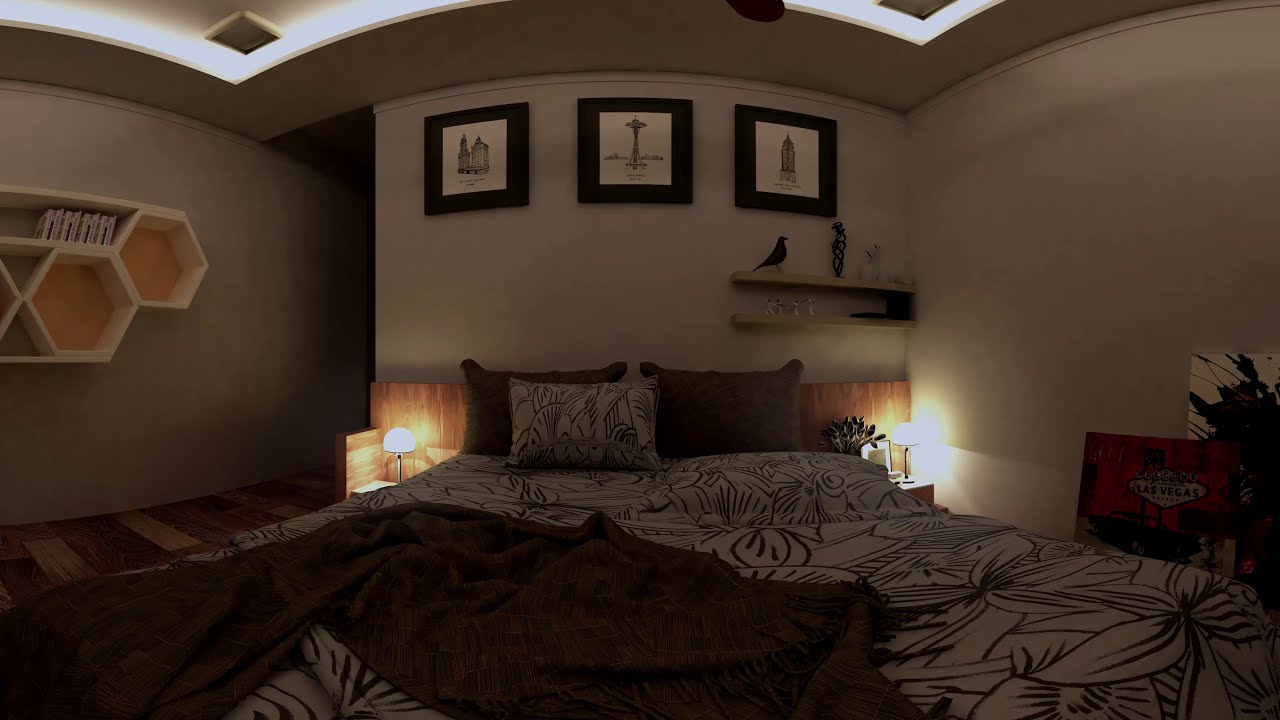The image features a dimly lit bedroom, with the perspective being from the foot of the bed looking towards the pillows. The room has beige-grayish walls and a light white ceiling with subtle backlit lighting adding a soft glow to the setting. High on the wall, almost where the ceiling begins, are three framed pictures of famous buildings, including the Empire State Building, the CN Tower, and the Tribune Tower in Chicago. Beneath these are a couple of shelves displaying various knickknacks and small sculptures.

The bed, positioned centrally in the room, has a wooden backrest adorned with small lights and a plant on each side. It is neatly arranged with three pillows—two brown and one white with a gray pattern. The white blanket features black lines forming floral patterns, adding a delicate touch to the bedding. Despite the overall dimness of the room, there is some minor lighting coming from both the left side, possibly from a table, and the right side, contributing to the ambiance that feels like it might be late at night.